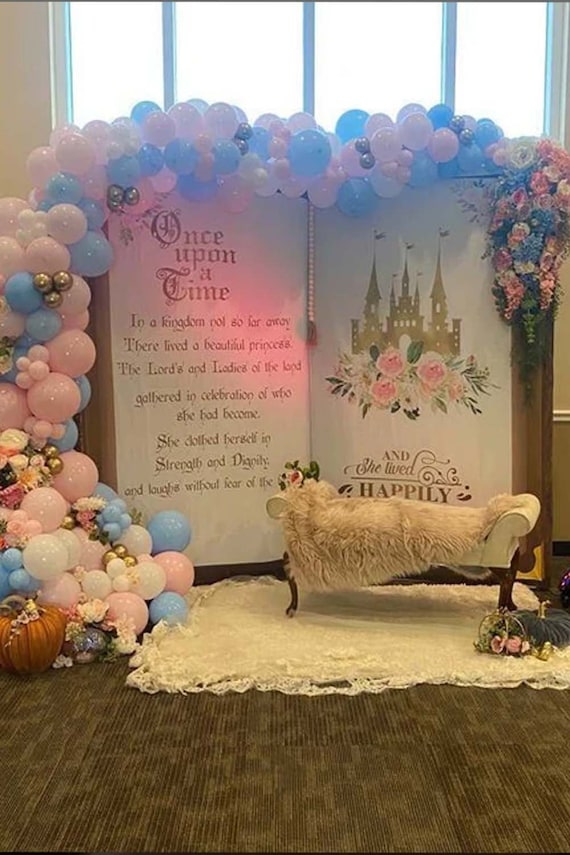The image depicts an indoor exhibit set up to resemble a fairy tale storybook scene, likely located in a reception hall or hotel lobby. The exhibit features a large open book partition with Gothic print text. On the left-hand page, it reads, "Once upon a time in a kingdom not so far away. There lived a beautiful princess. The lords and ladies of the land gathered in celebration of who she had become. She dolled herself in strength and dignity." The right-hand page includes an illustration of a castle and the phrase, "She lived happily ever after."

In front of the right-hand page is a cozy bench adorned with a fleece covering, placed on a white rug. Surrounding the book are clusters of balloons in shades of pink, white, blue, and gold, with some balloons inlaid with flowers. This area appears designed as a photo spot, giving visitors the opportunity to sit and immerse themselves in a whimsical, princess-themed setting.